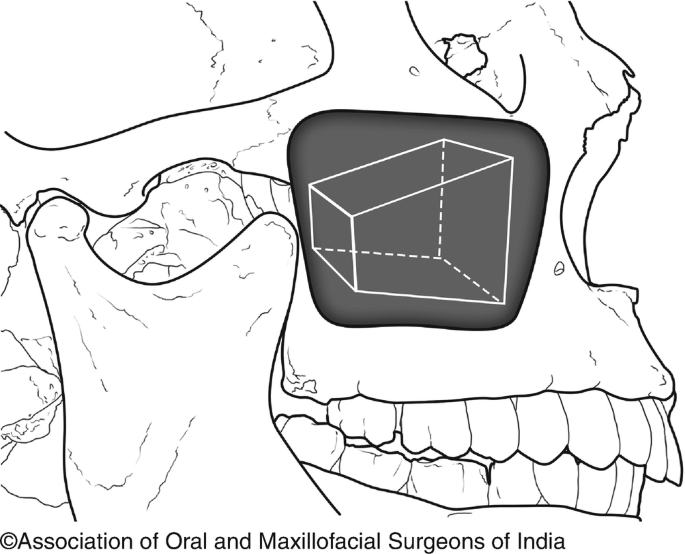The image depicts the right side of a large, intricately detailed skull, drawn in black on a white background. The skull features a clearly defined jaw and prominent front teeth. The eye sockets are asymmetrical and peculiar: the left eye is an oddly shaped gaping hole, while the right eye socket contains a three-dimensional black square with a smaller white square inside, marked by dashed lines indicating depth. The top of the skull, where the forehead should be, is also visible. On the left side of the image, there appears to be a giant bone or tooth-like structure. At the bottom of the image, there is text that reads "Association of Oral and Maxillofacial Surgeons of India," suggesting that this might be an illustrative rendition for educational or professional use. The entire drawing is outlined in black, but the central area remains pure white, contributing to the overall complexity and difficulty in distinguishing specific parts.